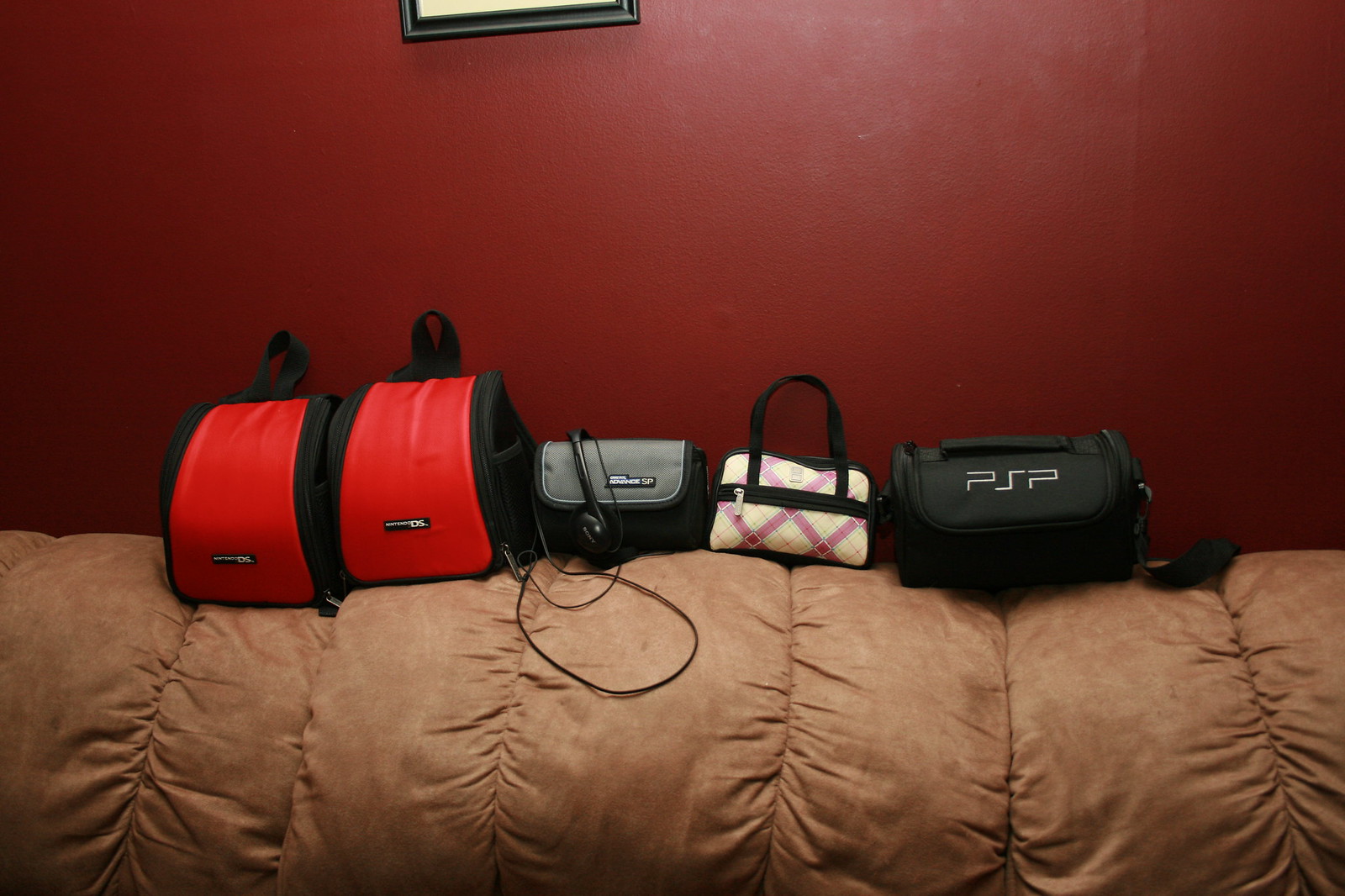The photograph captures a lineup of five bags resting on the back of a light brown couch, which is positioned against a deep red wall. The couch is divided into seven sections by visible stitching, adding a unique texture to its light brown fabric. Starting from the left, the first two bags are tall and identical, featuring large red stripes down their fronts, black sides, and small black loop handles on top. The middle bag is a small black satchel with a gray flap, adorned with an old pair of black headphones draped over it, with the cord trailing down. Beside it is a pink and purple plaid purse with black sides, a black handle, and a black zipper running across the center. The last bag on the right is a wide, black PlayStation tote bag prominently displaying the "PSP" logo in silver at the top. Above the couch, the rich red wall serves as a backdrop and features the edge of a black-framed picture.